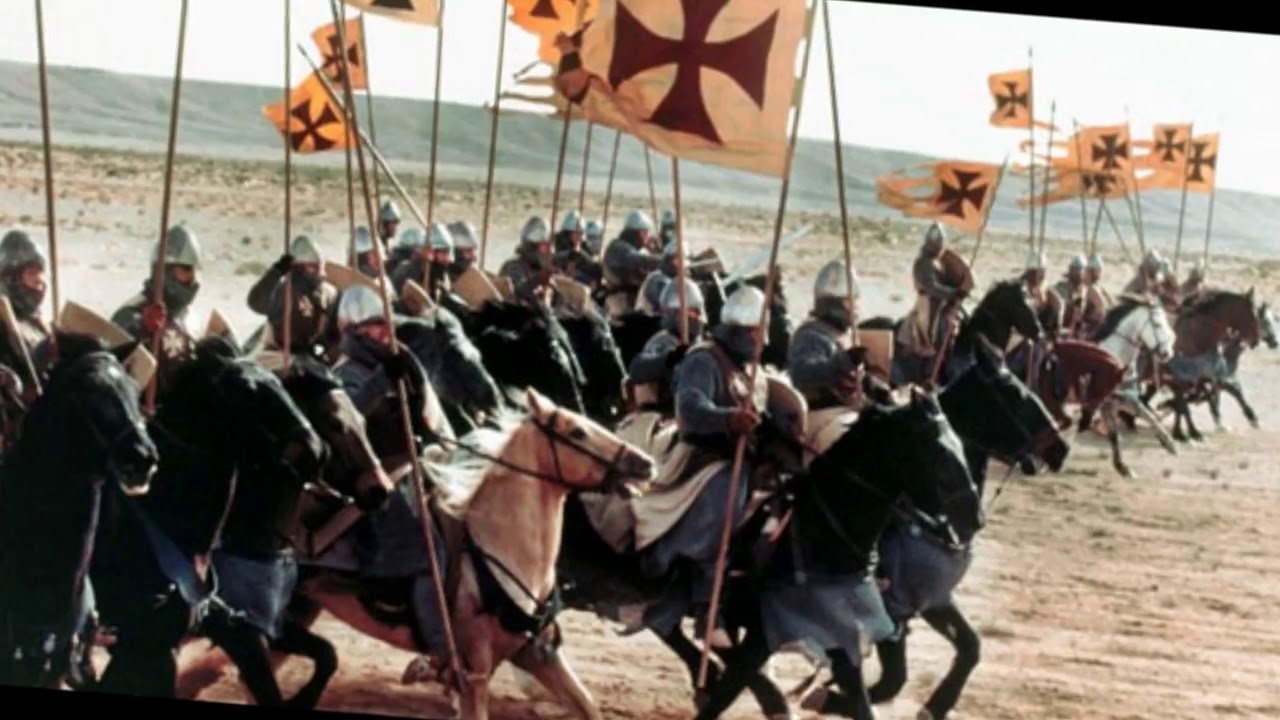This still from a movie depicts an intense medieval battle scene set in a desert landscape that stretches out for miles with minimal vegetation. The image shows a multitude of knights charging forward on horseback, suggesting a large-scale battle. The knights are clad in historical armor, including metal helmets and chain-link body armor covering their bodies and legs. They are armed with swords and spears, and each knight holds a banner that features a red cross on a white background, reminiscent of the Crusades. The cross design flares out at the ends and tapers toward the middle.

The horses in the scene vary in color, including black, fawn, palomino, and brown with white muzzles, adding to the diversity of the cavalry. The knights are seen riding in a structured formation, with the majority of the black horses clustered in the bottom left corner and a mix of light brown and white horses on the right side. The battle takes place on a dry, desert-like terrain with some hills visible in the background, reinforcing the harsh environment of the scene.

The image appears to be a photograph of a screen, possibly from an older film given the slightly washed-out quality, suggesting it might date back to the 1960s or 70s. This cinematic portrayal, possibly inspired by the Crusades or similar historical periods, vividly captures the chaos and grandeur of medieval warfare.